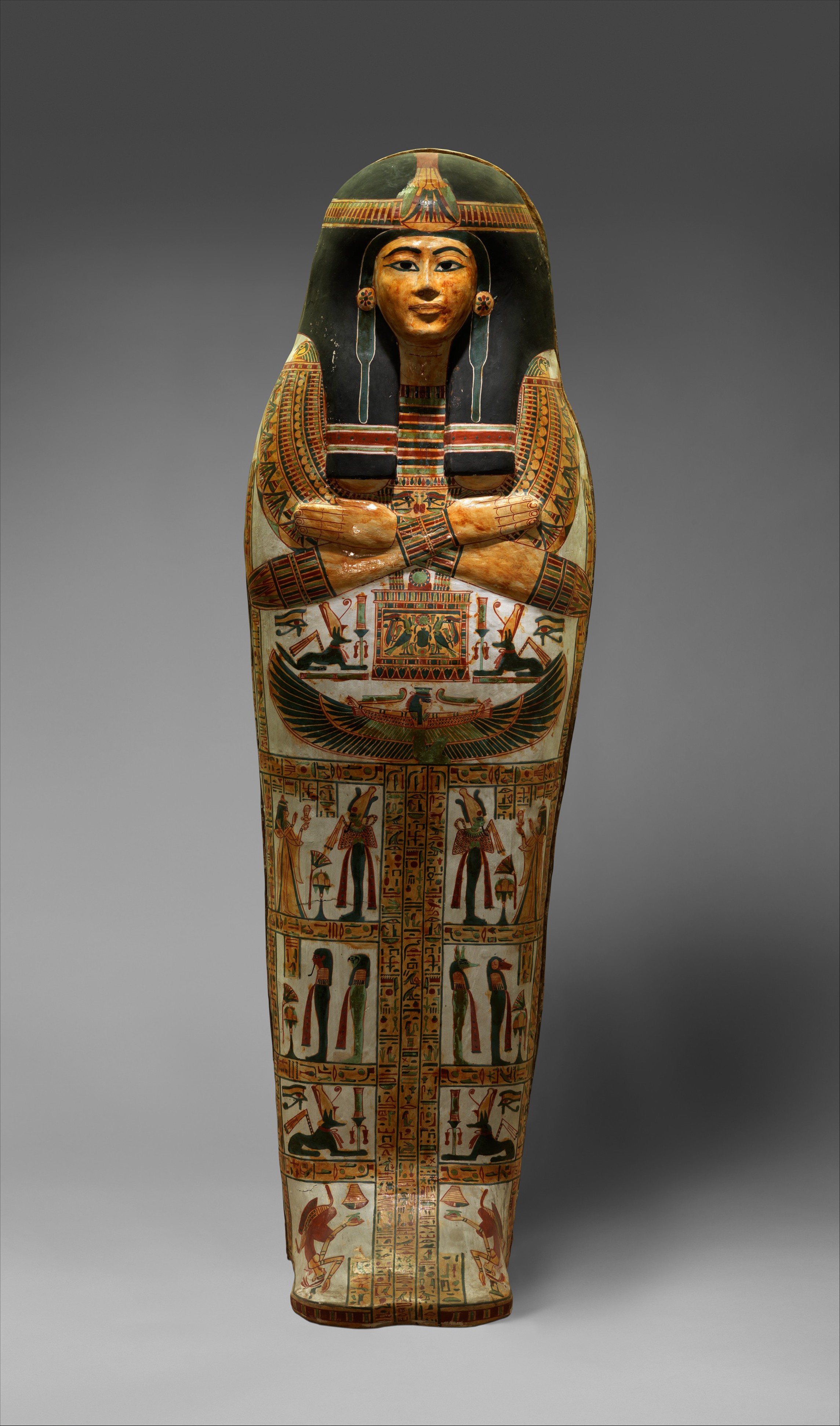In this photograph, we see a detailed, upright sarcophagus shaped like a pharaoh, typical of ancient Egyptian burial practices. The sarcophagus is predominantly brown with clear beige sections, and it features the face of a pharaoh with a long black crown of hair flowing down. The headwear includes a headband that goes across the top and around the head. The arms are crossed over the chest, a characteristic position, and the legs are together. 

Below the arms, the sarcophagus depicts two jackals sitting in front of an item. Around the stomach area, there is an illustration of an Egyptian boat, seemingly resting in front of a temple. The sarcophagus is adorned with various other markings and drawings, including depictions of Egyptian gods holding objects. Along the lower half, small figures and symbols suggest themes of loyalty and companionship in the afterlife. The warm, earthy tones and intricate design elements, including people and animals, reflect a rich cultural heritage, enhancing the sarcophagus’s attractive and storied appearance.